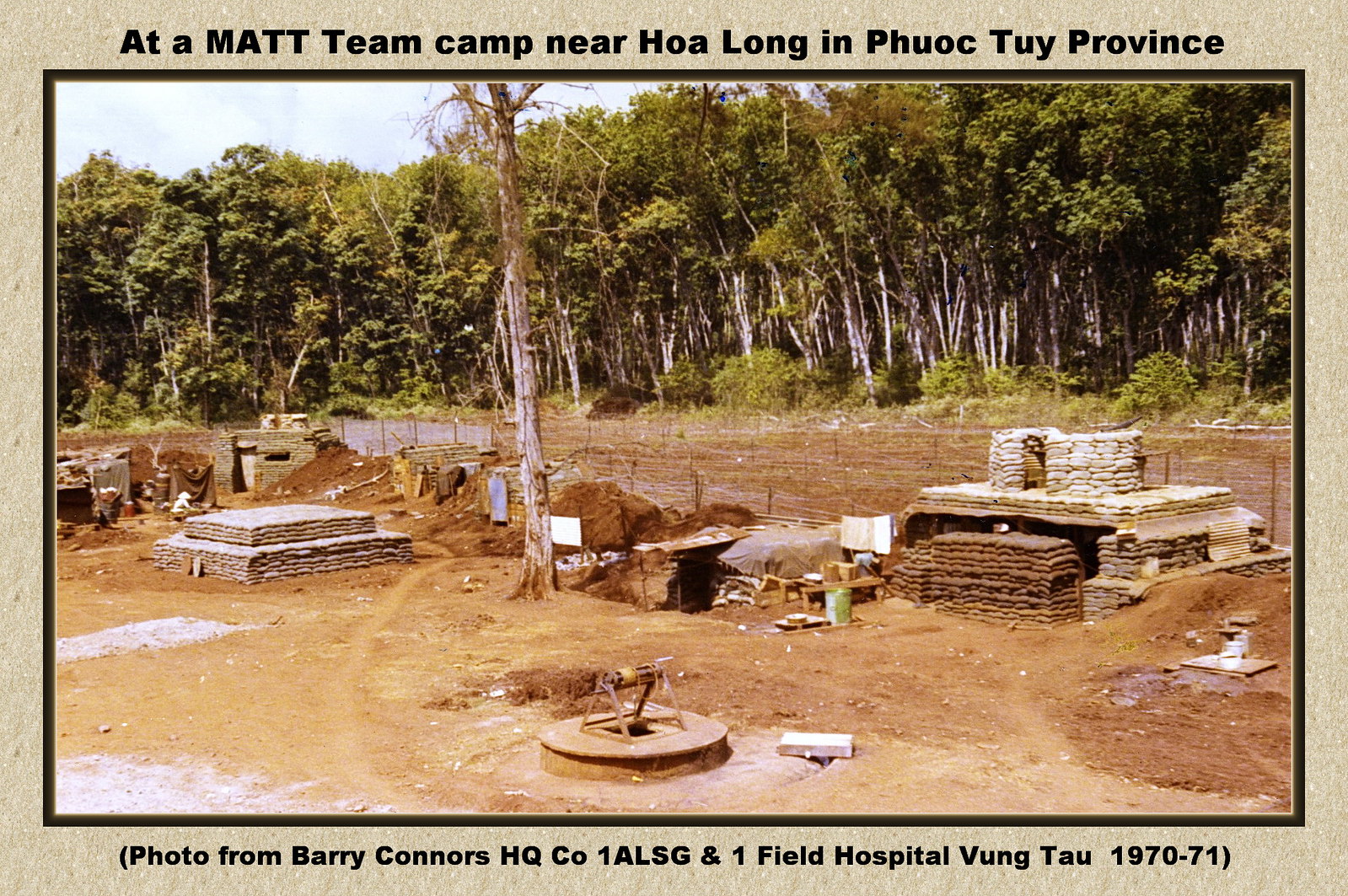This photograph, bordered by a thin, dark line and an outer light sandstone brown edge, captures a rustic outdoor scene set within a larger forested area. In the foreground, an expanse of plowed dirt is partially enclosed by makeshift fences. Prominently, a slightly dead-looking tree stands in the center, surrounded by various structures. One of these structures is a hut made of sandbags, appearing as if it has been burrowed into the ground. Adjacent is a recently constructed well with a rope extending into it, likely holding a bucket. Nearby, another sandbag structure resembling a stand is visible, accompanied by additional sandbag constructions featuring small windows and doors.

The upper portion of the photograph showcases a dense row of lush green trees against a backdrop of blue sky. Behind the main scene, a road has been carved out along the forest's edge. The photograph is an archival image from Barry Connors, HQ Co., 1ALSG, and Onefield Hospital, Vung Tau, 1970-71. The captions at the top and bottom of the image read, "At a MATT team camp near Hoa Long in Phuoc Thuy province." This detailed snapshot offers a glimpse into the rudimentary living conditions and ongoing construction efforts within an army barracks setting from the Vietnam War era.